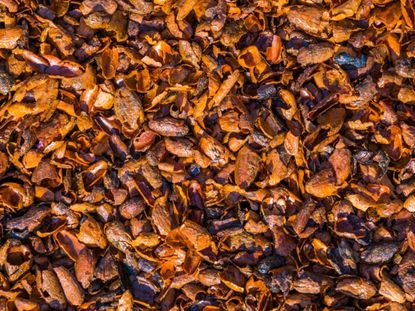The photograph depicts a close-up of an area densely covered with an array of curled, crunchy-looking objects in various shades of brown, ranging from burnt orange to reddish and cool tones. The texture and shapes are reminiscent of peanut shells or dried leaves, twisted and hollow like cocoons. The objects are scattered uniformly across the scene, evoking the appearance of a natural forest floor littered with these elements. Some areas suggest the presence of mushrooms or bark, adding to the complexity of the textures. The image is so zoomed in that it becomes challenging to definitively identify what's depicted, leaving an impression of a chaotic and richly detailed landscape. One might even glimpse unusual shapes, such as something resembling the head of a snake in the upper left-hand corner, contributing to the enigmatic and textured atmosphere. If you stepped on these objects, they would likely make a satisfyingly crunchy noise.